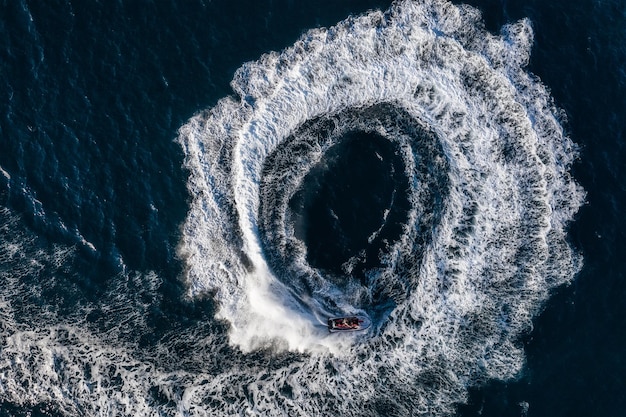This is a color photograph captured from a high vantage point, likely a drone, providing a bird's-eye view of a jet ski creating an impressive circular wake in the dark blue ocean. The image features a jet ski near the bottom of a large, swirling white ring of foam, positioned at about six o'clock if the circle were viewed as a clock face. The wake forms a perfect ring, resembling a bullseye or target, accentuating the dynamic motion and spiraling energy of the scene. The jet ski appears to have started its path from the bottom left corner before maneuvering into this striking circular pattern, with water visibly spraying up from its rear. The entirety of the frame is filled with the contrast between the dark, almost black ocean and the bright, roaring white ring of the jet ski's wake. This detailed and dramatic composition underscores the swift and skillful movement of the jet ski amidst the vast expanse of the sea.